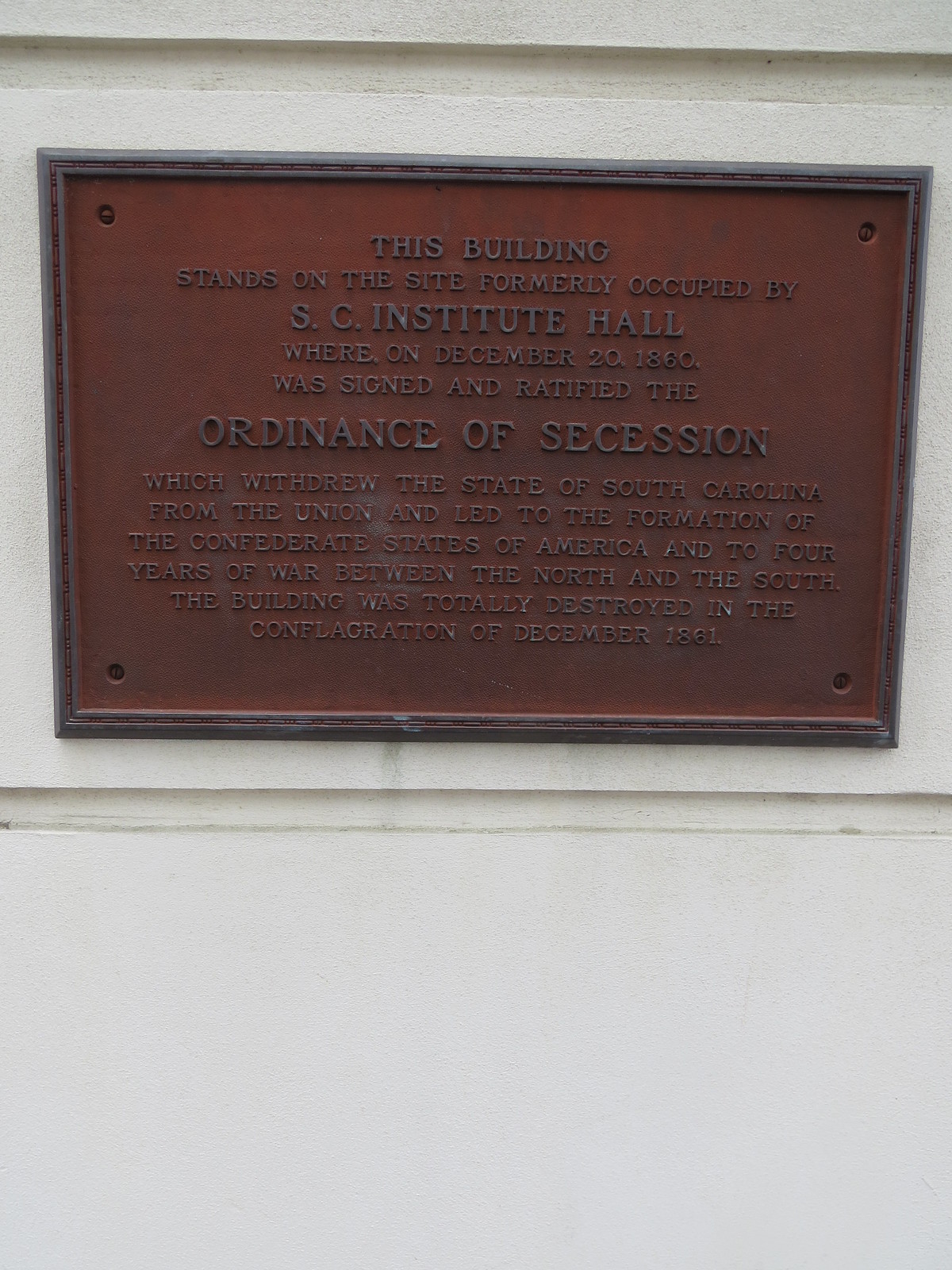The image depicts a weathered iron placard with a rusty red hue and a gray border, securely mounted by flathead screws at each corner to a solid white stone or granite wall. Despite its age and worn appearance, the raised text on the placard remains legible. The inscription reads: "This building stands on the site formerly occupied by SC Institute Hall, where on December 20, 1860, was signed and ratified the Ordinance of Secession, which withdrew the state of South Carolina from the Union and led to the formation of the Confederate States of America and to four years of war between North and South. The building was totally destroyed in the conflagration of December, 1861."